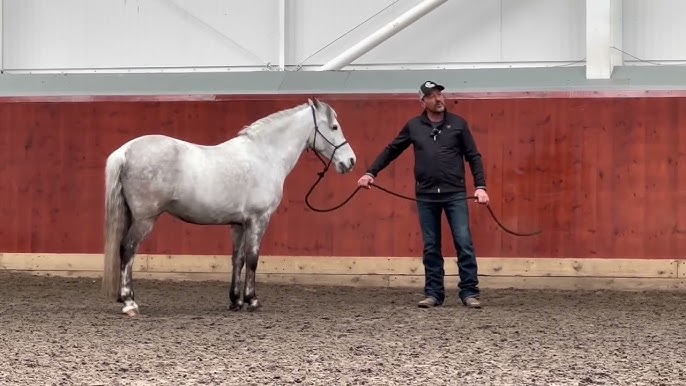In this detailed photograph, a man stands holding a leash attached to a distinctive horse, which could be a smaller version of a Lipizzaner stallion. The horse itself is mostly white with gradients of gray and brown on its legs and towards its tail. The man is positioned on the right and is dressed in a black jacket, dark blue jeans, and a black cap. Behind them, there's a red painted wooden structure, the bottom part of which is brown, and there are visible pipes against a white section of the wall above the red facade. They are standing on a dark gray, soil-covered ground, suggesting a stadium or training environment. The man is holding the black leash with both hands, wrapped around the horse's muzzle, indicating a scene of training or handling. There are no texts visible in the image.